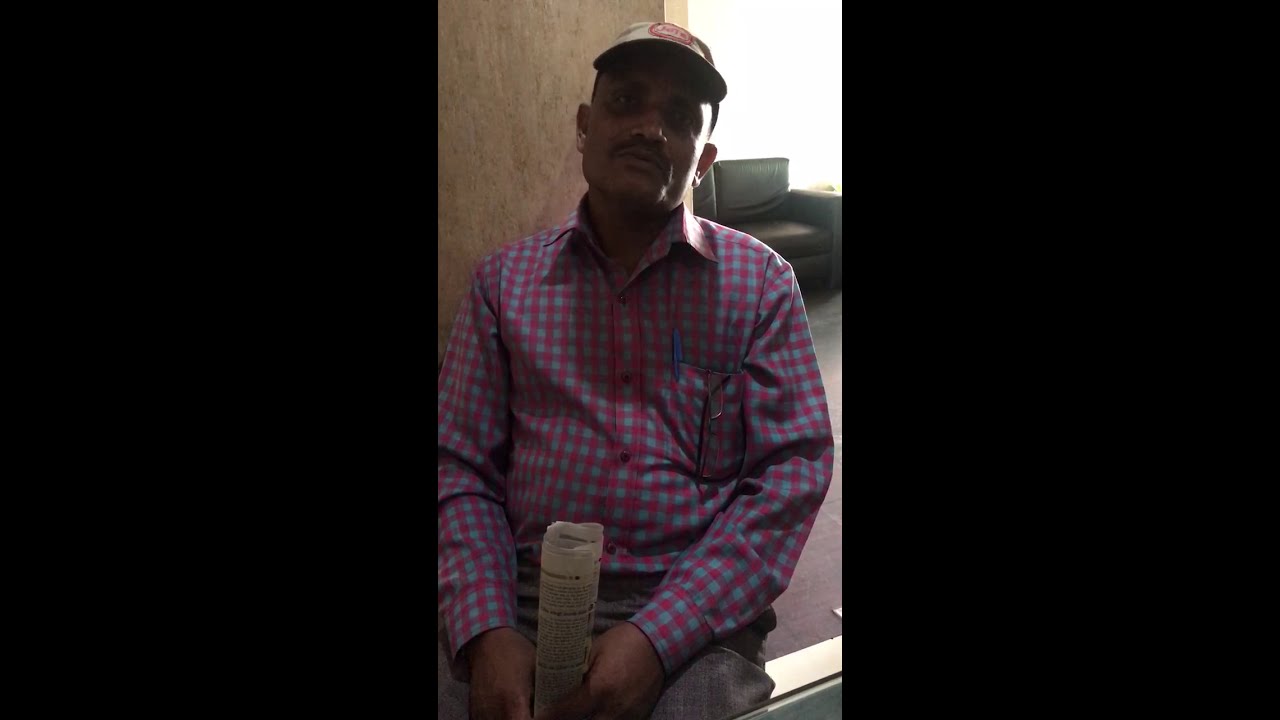In the center of the photograph, framed by black vertical strips on either side, sits a middle-aged man of dark to medium skin tone. He wears a red and blue plaid checkered long-sleeve shirt with a blue pen cap clipped in the chest pocket and gray pants. A tan baseball cap with a red disc logo adorns his head. The man, with a thin mustache and a slightly bored or sad expression, leans slightly back and to the right. He holds a rolled-up newspaper between his hands, which rest between his legs. The background features a wall, an open doorway leading to another room with sunlight streaming in through a window, and a dark sofa or couch. Subtle details like the light hitting the left side of his face and various furnishings suggest a casual indoor setting.